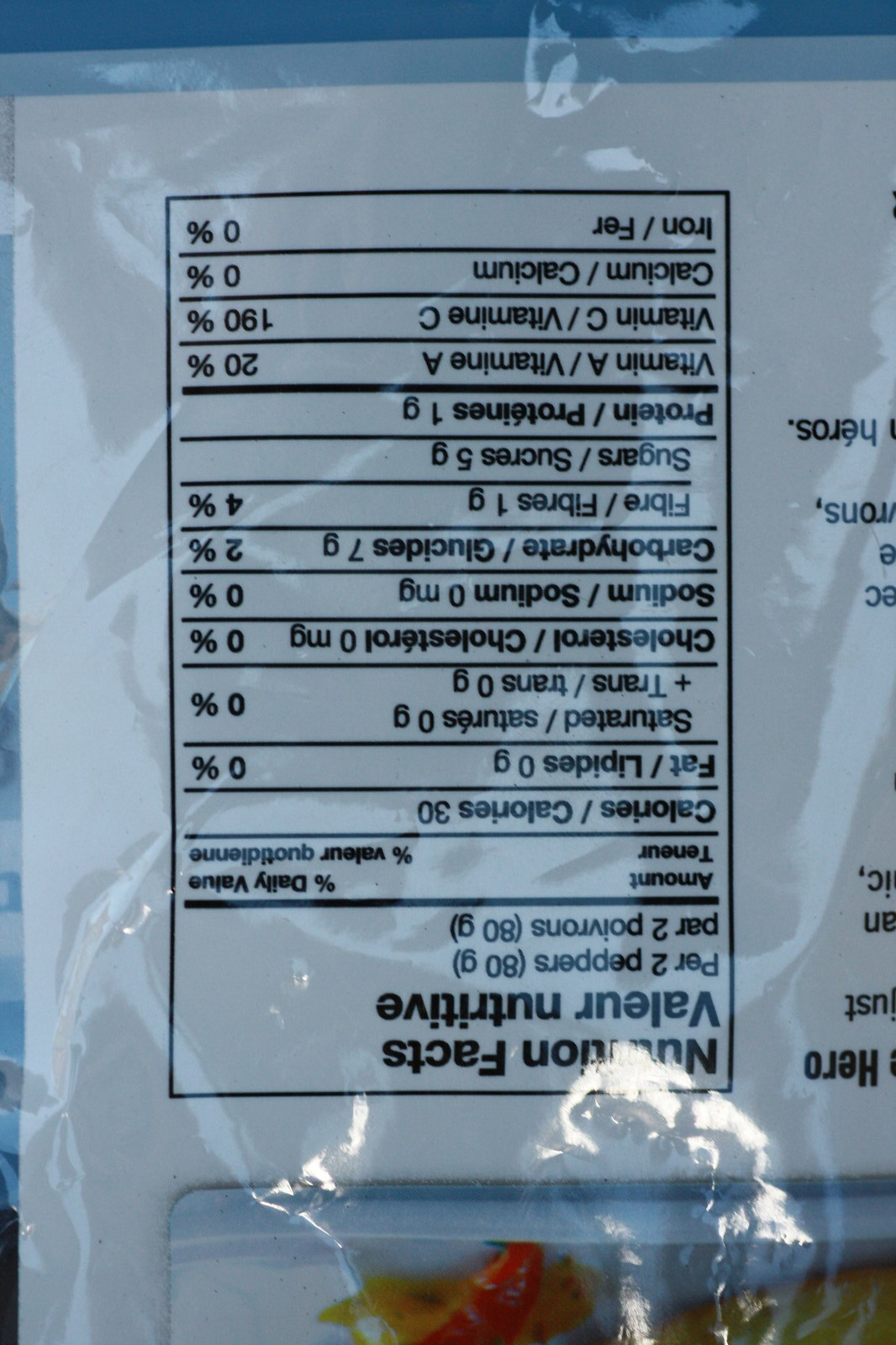This upside-down image captures the back of a frozen food item, focusing primarily on the nutritional facts section. Despite the orientation, the details are discernible. The nutritional label indicates that the product contains no fat, saturated fat, cholesterol, or sodium. It provides 2% of the daily value of carbohydrates per 7 grams, 4% of dietary fiber, 20% of vitamin A, and a remarkably high 190% of vitamin C. The product has no calcium or iron content. Given these nutritional details, it's likely that this is a frozen vegetable or possibly a frozen meat product enriched with vitamins.